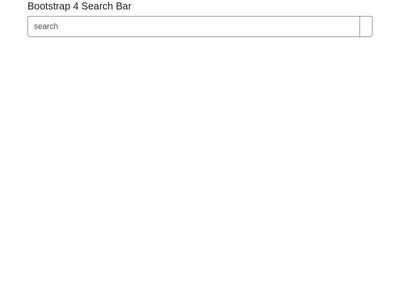The image showcases a minimalist, mainly white background with black text at the top. On the left side of the page, it reads "Bootstrap 4 Search Bar." Dominating the page is a long, light gray search bar that spans approximately 95% of the page's width. Inside this search bar, the word "search" is typed in lowercase, light gray letters. At the far right end of the search bar, occupying the remaining 5% of its length, is a small, gray rectangle with a white interior. The rest of the page below the search bar remains completely white, maintaining the clean and simple aesthetic of the overall design.